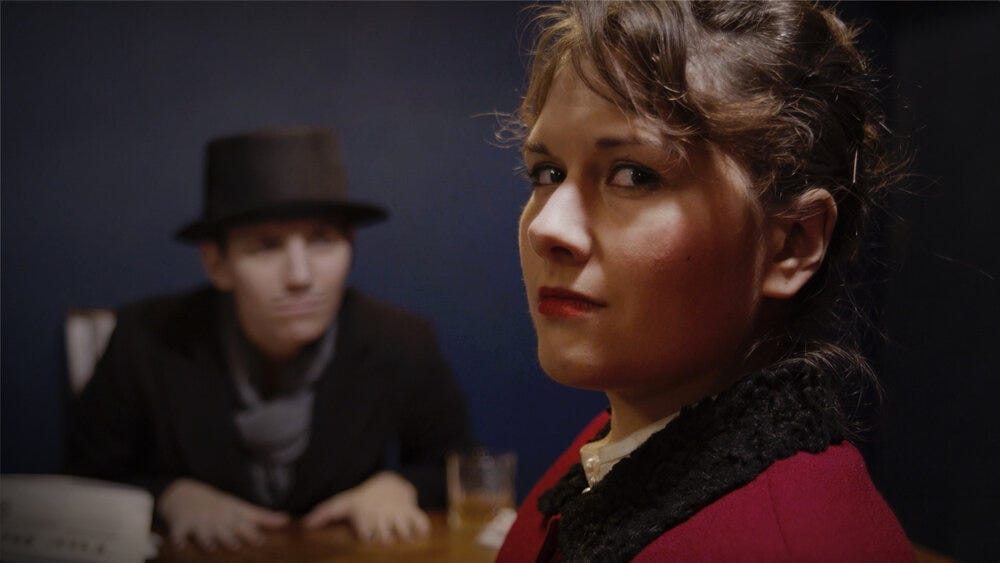In this horizontal rectangular image, two people are depicted against a very dark background. The woman on the right side of the image stands facing sideways, but her head is turned toward the viewer. She has brown, wavy hair pulled up with some strands hanging loose, secured with black clips. Dressed in a striking red suit with black fur trim around the collar, she also wears a high-collared white shirt with pearl buttons underneath and red lipstick. Shadows from her hair fall across her face, adding to the photograph's dramatic ambiance.

Further back on the left side, a man sits at a round brown table, with both hands placed palm down on its surface. A whiskey glass filled with amber-colored liquid is in front of him. He is dressed in a black coat, a gray neckerchief, and a black fedora. He also sports a thin, penciled-in black mustache. Although the man appears smaller and slightly blurry, he gazes toward the woman with an attentive expression. He is seated in a wooden chair, anchoring the scene's composition.